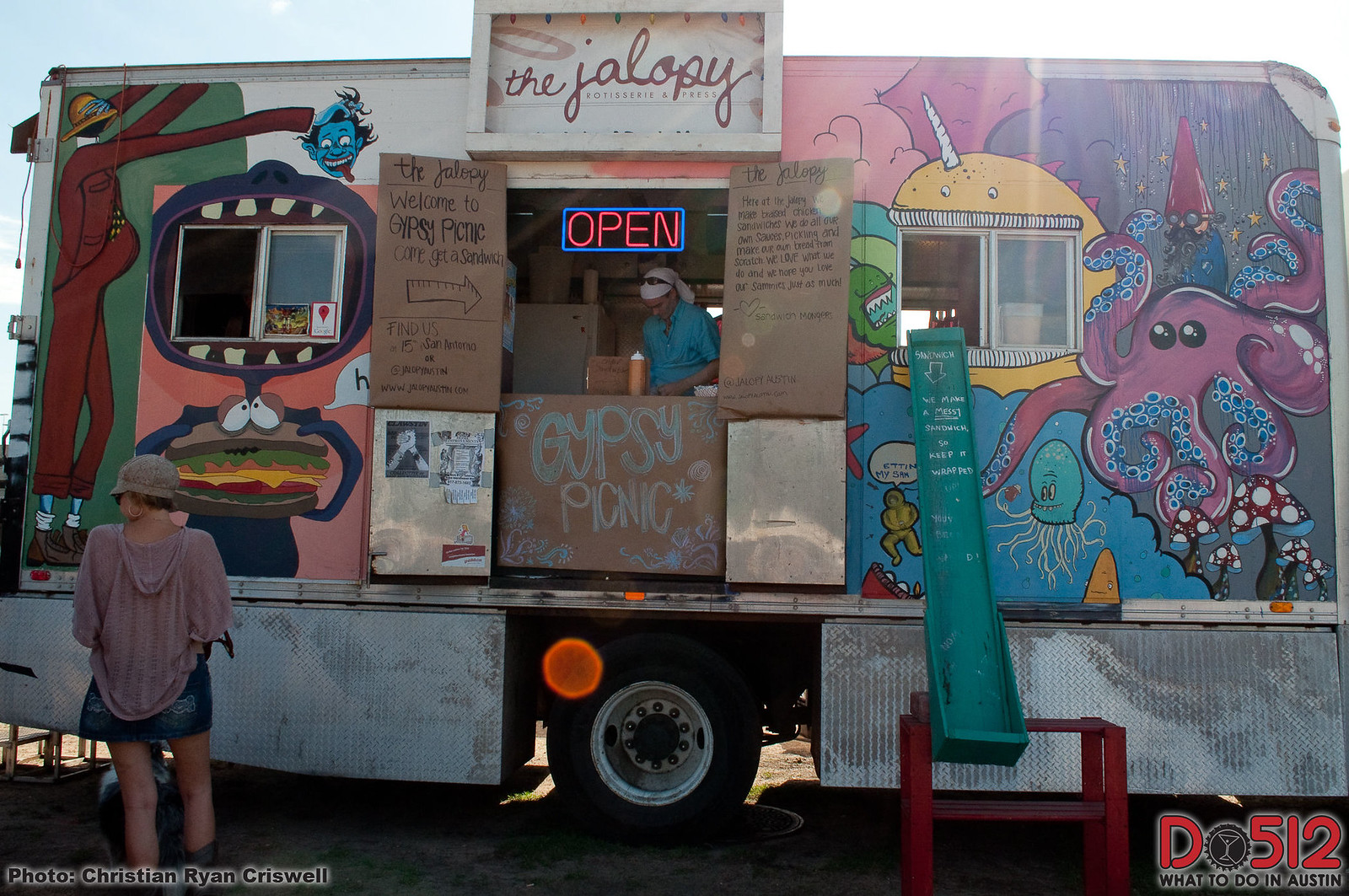This outdoor photograph captures a vibrant food truck named "The Jalopy" stationed at a location labeled "Gypsy Picnic." The truck is eye-catching, adorned with diverse and comical cartoon-like illustrations. On one side, a gigantic green woman resembling a tree with elongated arms and no hands, appears to be pregnant, wearing an oversized green hat. Nearby, a blue-skinned man with black hair, pointy ears, and a tongue sticking out, adds to the whimsical charm.

Moving to the right, a narwhal (a unicorn-like whale), a jellyfish, and a playful pink octopus are engaging visuals, alongside poisonous mushrooms with red caps and white spots. The left side features another purple octopus sporting a wizard hat, glasses, and a mustache.

Beneath these fantastical images, several text signs are visible. A prominent neon "open" sign marks the ordering window, where a man wearing a turquoise blue shirt and a white headscarf attends to customers. Just below, a cardboard sign reads "Gypsy Picnic" and another states, "The Jalopy - Welcome to Gypsy Picnic." Additional text mentions their specialty in making brisket chicken sandwiches, custom sauces, pickling, and homemade bread, describing them as "hot sandwich mongers."

In the foreground, a woman dressed in a hat, purple shirt, and a short denim skirt stands near the food truck. The logo "D-O-512" indicating "What to do in Austin" is visible in the bottom right corner. The truck's quirky art and friendly service suggest a lively, welcoming atmosphere.